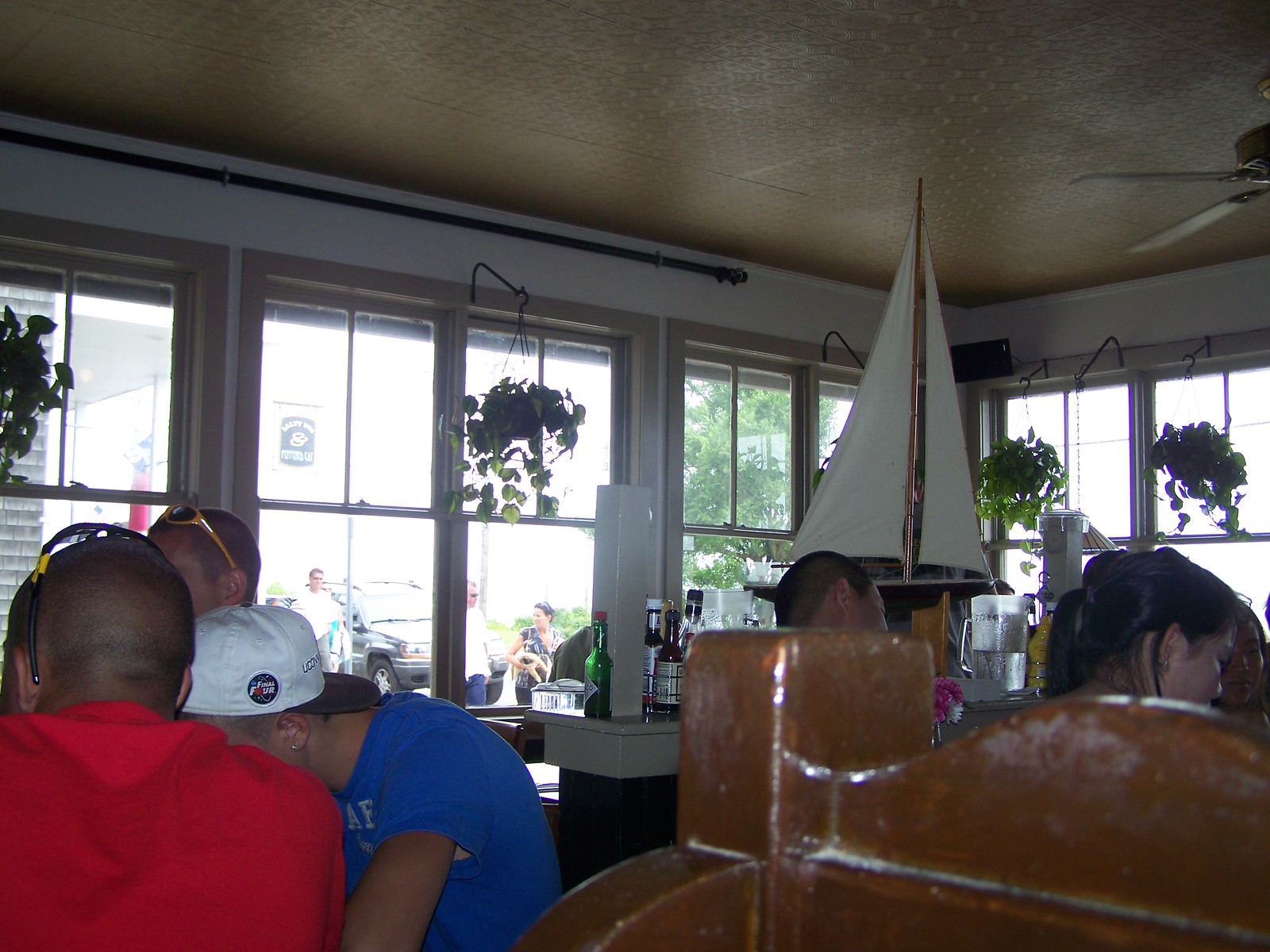The photograph captures the dynamic, lively interior of a cafe or restaurant. The room is adorned with bold-colored walls and features numerous windows that allow bright white light to pour in, revealing the lush greenery and trees just outside. Several cars and people can be spotted through these windows, and hanging baskets with vibrant green plants add a touch of nature to the decor.

Inside, the left side of the image shows three men seated in a group. One is wearing a red T-shirt, another is in a blue T-shirt with his back turned, and a third man in the background sports sunglasses perched on his head and a baseball cap. The right side of the image includes additional patrons and a glimpse of a wooden post or booth near the bottom right corner.

A notable feature is a model sailing ship situated in the center-right of the image, with triangular white sails and a black body, adding a nautical theme to the ambiance. The ceiling hosts a fan on the top right side, contributing to the home's comfortable environment. Classic restaurant condiments—a green Tabasco bottle and a white A1 steak sauce bottle—are visible, enhancing the authenticity of the dining experience. Overall, the photograph exudes a bustling, cozy atmosphere perfect for social gatherings.